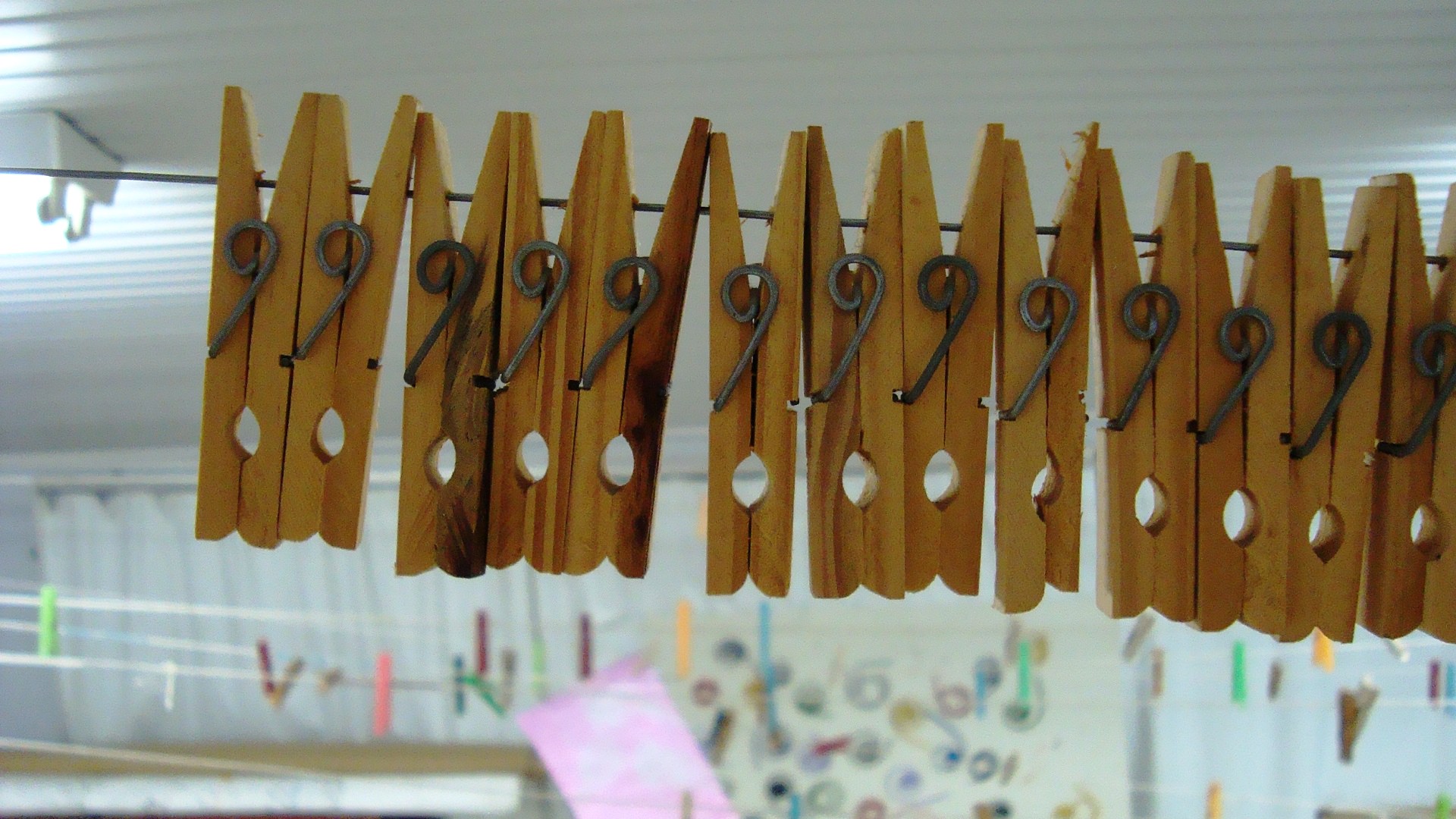The photograph is a horizontal rectangular image featuring a close-up view of traditional wooden clothespins suspended by their pinchers from a wire. Each clothespin has a tiny hole drilled through the top part to accommodate the wire, and they are arranged side by side, showcasing a mix of natural wood tones with some darker and lighter spots. The wire goes horizontally across the top third of the photograph. The background reveals a white or light gray ceiling with some striped or tone-on-tone details, and light shining from the upper left corner. Behind the primary wire, multiple other lines with clothespins—made from colored plastic in hues like pink, maroon, green, light green, and blue—hint at an art room setting. Additionally, a blurred background features what seems to be another project with items hanging on a whiteboard, and a piece of pink paper tilted slightly toward the right bottom corner adds to the artistic ambiance.